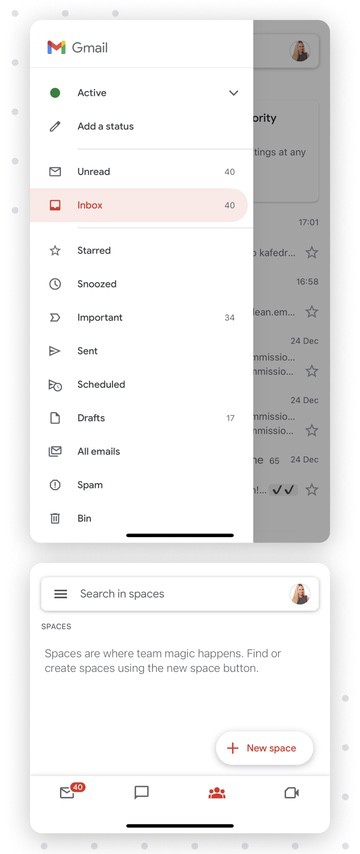A detailed screenshot of a mobile phone app webpage, likely displaying the Gmail interface. At the top, there is a white header featuring a vertical drop-down menu. On the left side of the header, the word "Gmail" is displayed, accompanied by a small "M" Gmail icon to its right. Below this header, a vertical list is visible, comprising various labels and categories. These include "Settings," "Active," "Out of status," "Unread," "Inbox" (which is currently selected), "Starred," "Snooze," "Important," "Sent," "Scheduled," "Drafts," "All emails," "Spam," and finally "Bin." Each item in this list is paired with a corresponding icon on its left side.

Beneath the list of labels, there is a white search box labeled "Search in spaces." Below this search field, the text "Spaces are where Team Magic happens. Find or create spaces using the new space button." is displayed. Following this text, a prominent button with red text and a plus sign next to it reads "New space."

At the bottom of the screenshot, four icons are lined up horizontally: an envelope icon with a red badge indicating 40 unread messages, a speech bubble icon, and an icon of a crowd of people.